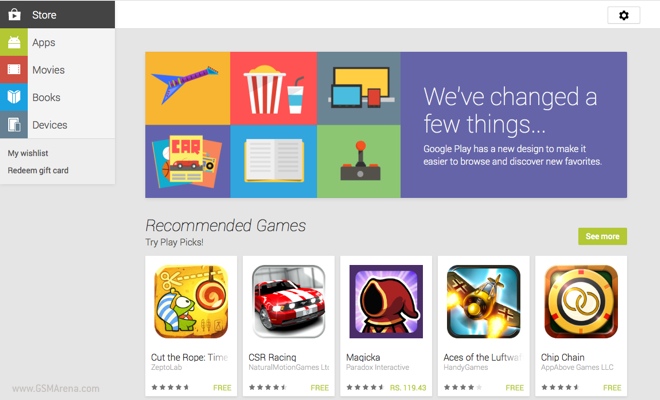### Detailed Caption for a Screenshot

This image is a screenshot from an app store interface, likely the Google Play Store. The layout is divided into several sections. On the left-hand side, there is a vertical menu with the following categories listed from top to bottom: "Store", "Apps", "Movies", "Books", and "Devices". Beneath these primary sections, in smaller print, are additional options: "My Wishlist" and "Redeem Gift Card".

At the very top of the interface, there is a white navigation bar. Positioned in the top right-hand corner of this bar is a Settings button.

Below the white navigation bar, there is a colorful photo collage consisting of a few illustrations: an electric guitar, a popcorn and drink combo, a TV, tablet, and phone screen, a stack of books or magazines, an open book, and a game joystick. Adjacent to this collage, a message reads, “We've Changed a Few Things. Google Play has a new design to make it easier to browse and discover new favorites.”

Further down, the page presents a section titled "Recommended Games". Under this heading, a subheading reads "Try Play Picks". The games listed here include "Cut the Rope", "CSR Racing", "Magica", "Aces of the Luftwaffe", and "Chip Chain". At the bottom of the list, there is a button labeled "See More" that presumably allows users to view additional game recommendations.